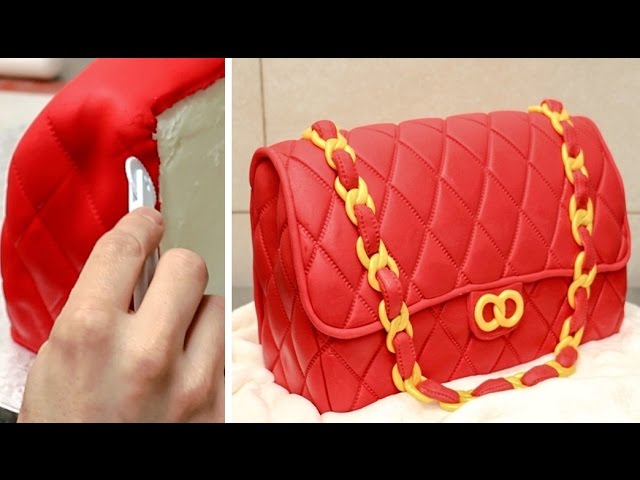This image features a handcrafted cake meticulously designed to resemble a red leather patent purse, displayed through two side-by-side photographs. On the left, a Caucasian hand is seen using a miniature plastic pastry wheel to imprint diamond patterns onto the cake's red fondant cover, simulating the detailed texture of leather. The right photograph showcases the completed, realistic purse cake, set against a soft, plain towel background. The edible purse boasts a solid red color except for its strap—a gold chain interwoven with a red strap—draped elegantly over it. The purse also features two interlocking gold circles resembling the Olympic rings on the front, presumably representing the branding of the purse.